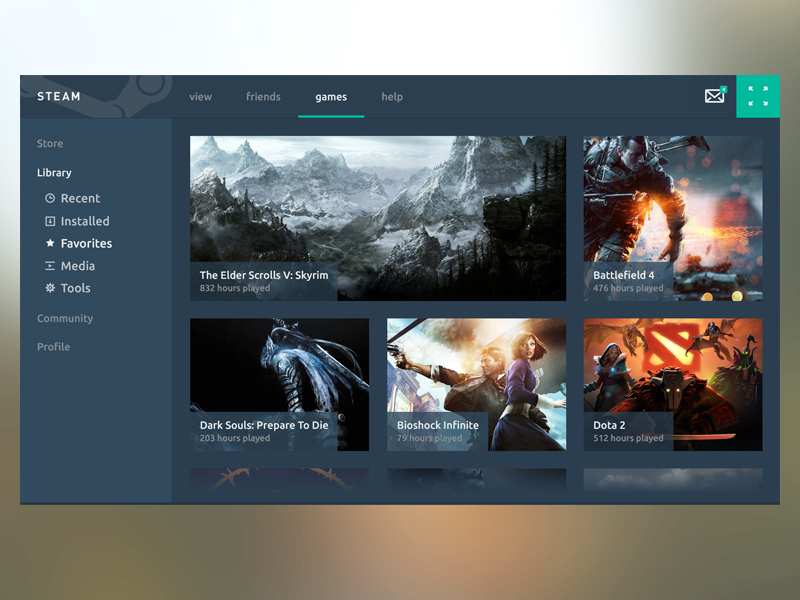A screenshot of a digital storefront interface is displayed. At the top, the heading "Steam" is prominently featured. The interface includes a left-hand navigation bar with tabs labeled: Store, Library, Recent, Installed, Favorites, Media, Tools, Community, and Profile. Centrally located, additional navigation options read: View, Friends, Games, Help. Below these, five video thumbnails or game icons are arranged in a row. The listed titles are: "The Elder Scrolls V: Skyrim," "Battlefield 4," "Dark Souls: Prepare to Die Edition," "BioShock Infinite," and "Dota 2," each showcasing distinctive visuals. The collection appears to consist mainly of popular action-adventure and role-playing games, suggesting a selection of animation-based gaming content.